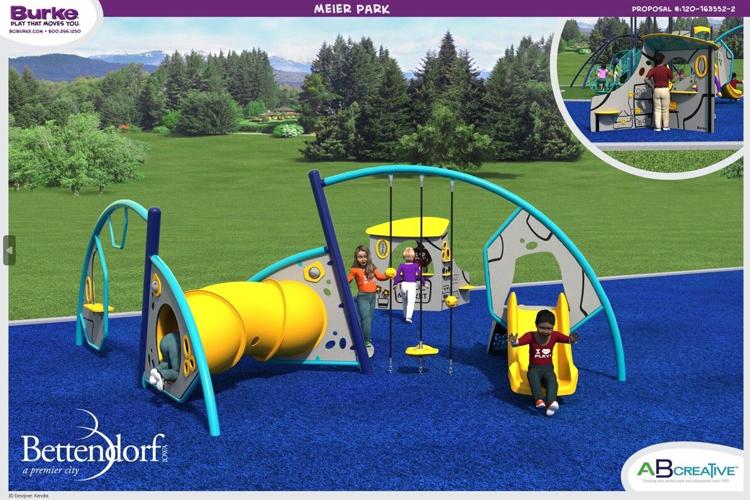This is a digitally designed horizontal rectangular image, reminiscent of a video game, featuring an advertisement for a children's playground. The upper section showcases a large expanse of green grass, tall pine trees, a cloudy sky, and outlines of mountains in the background, all under a purple border. Centered in the purple border, the text "MEIER PARK" is prominently displayed in all caps, with the brand "Burke" and the tagline "Play That Moves You" inside a white oval on the upper left side. The upper right corner features a telephone number for proposals.

The main image depicts a brightly colored playground set against a blue turf floor that contrasts against the green grass. The playground equipment includes a yellow tunnel, blue arches, poles, and a small yellow slide. Four children can be seen playing; one child is partially visible entering the yellow tunnel, another is going down the slide, an African American boy is on the side, and there's a supervising adult, possibly a mom. 

The lower-left corner of the image has the text "Bettendorf" in white letters, while the lower right corner displays "AB Creative."